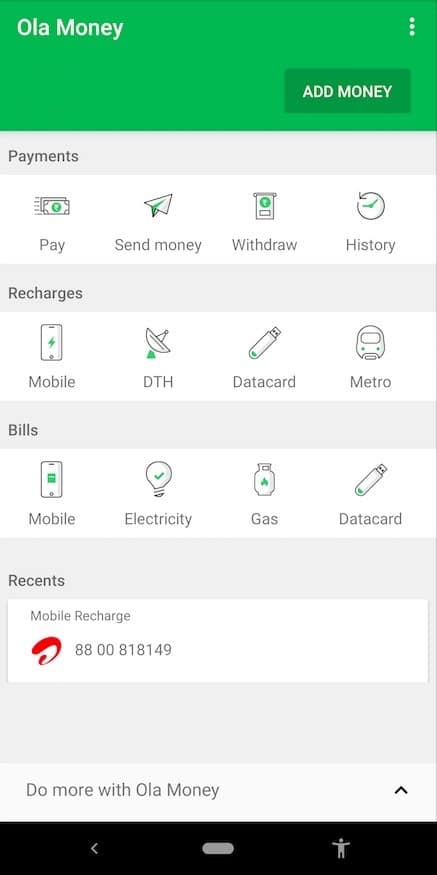Here is a descriptive and detailed caption based on the provided information:

---

Screenshot of the Ola Money app displayed on a mobile screen. The app is characterized by a simple and clean design. At the top, there is a green header with "Ola Money" written in white text, without any logo. On the far right of the header are three vertically-aligned dots, typically indicating a menu or settings option.

Below the header is a darker green button with white text that reads "Add Money." The main screen background is light gray, segmented into different categories divided by white horizontal sections.

The categories, listed in dark to medium gray text, include:

1. **Payments**: Contains options such as "Pay," "Send Money," and "Withdraw History."
2. **Recharges**: Includes "Mobile," "DTH," "Data Card," and "Metro."
3. **Bills**: Lists "Mobile," "Electricity," "Gas," and "Data Card."
4. **Recents**: Displays a recent mobile recharge transaction with the number "8800-818-149."

At the bottom of the categories section is a white box titled "Do More with Ola Money," accompanied by an up-pointing arrow, likely to expand or reveal additional information.

The bottom section of the screen resembles a typical phone's navigation bar, featuring a black background with lighter gray icons.

---

This caption provides a clear and detailed description of the Ola Money app's interface based on the provided voice description.